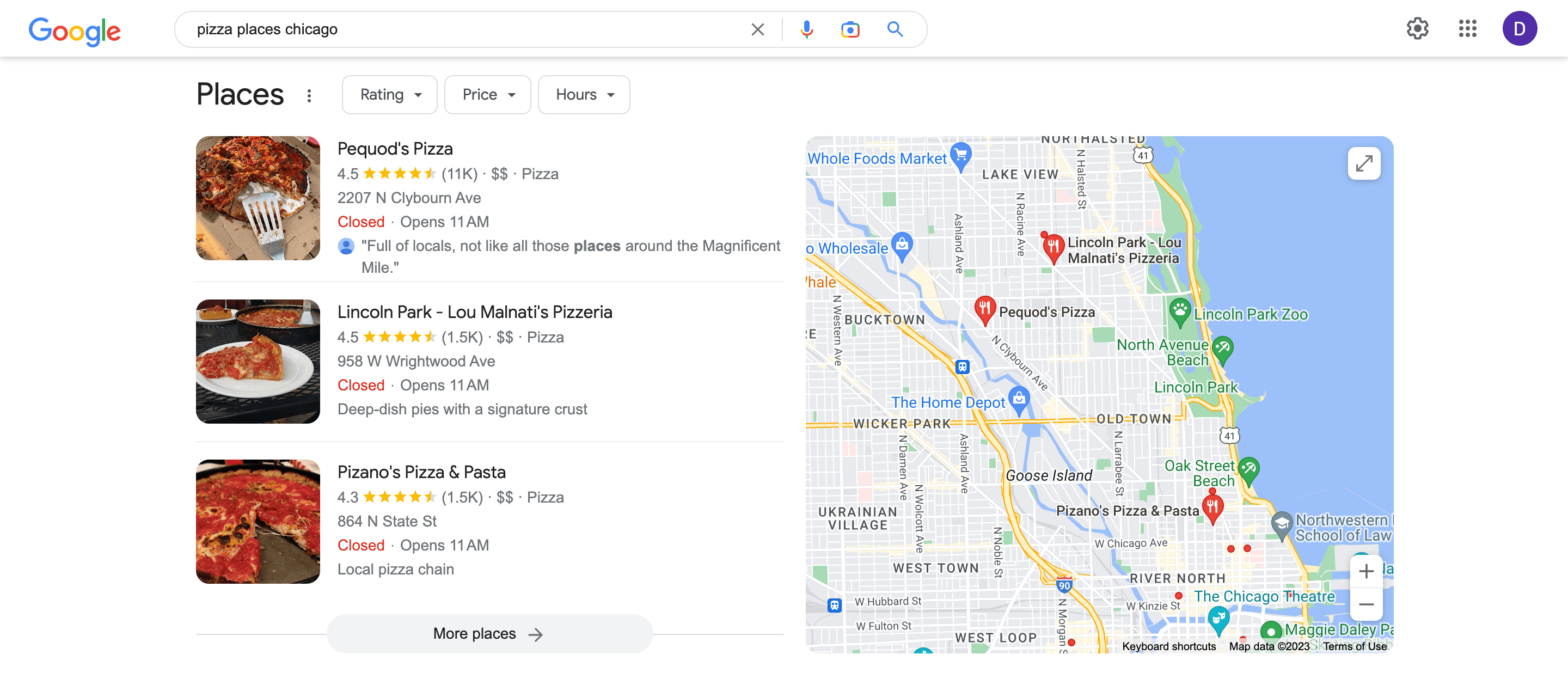The image displays the results of a Google search for "Pizza Places Chicago." The interface includes icons for a microphone, a camera, and a magnifying glass positioned alongside the search text box. The results are presented in a list format with sorting options for rating, price, and hours at the top.

1. **Pequod's Pizza**
   - **Image**: A whole pizza on a spatula.
   - **Rating**: 4.5 stars based on 11,000 reviews.
   - **Price**: $$ (Moderately priced)
   - **Cuisine**: Pizza
   - **Address**: 2207 North Clybourn Avenue
   - **Hours**: Currently closed, opens at 11 AM.
   - **Comment**: Popular with locals, unlike many places around the Magnificent Mile.

2. **Lincoln Park Lou Malnati's Pizzeria**
   - **Image**: A single slice of pizza on a white plate.
   - **Rating**: 4.5 stars based on 1,500 reviews.
   - **Price**: $ (Inexpensive)
   - **Cuisine**: Pizza
   - **Address**: 958 West Wrightwood Avenue
   - **Hours**: Currently closed, opens at 11 AM.
   - **Comment**: Known for deep-dish pizza with a signature crust.

3. **Pizano's Pizza and Pasta**
   - **Image**: A pizza with one slice taken out.
   - **Rating**: 4.3 stars based on 1,500 reviews.
   - **Price**: $$ (Moderately priced)
   - **Cuisine**: Pizza
   - **Address**: 864 North State Street
   - **Hours**: Currently closed, opens at 11 AM.
   - **Comment**: A local pizza chain.

Below these entries, there's a "More places" button to explore additional options. On the right side of the image, a large map highlights the locations of these restaurants.